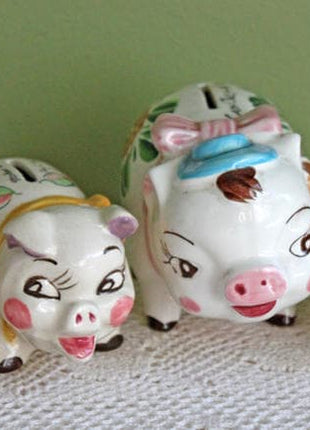This close-up photograph showcases two vintage, ceramic piggy banks, likely found on eBay or Etsy, placed on a white crocheted doily. Both banks are painted white with detailed facial features, and they vary in size. The larger piggy bank, situated on the right, sports a blue hat with a tuft of brown hair beneath it, thin long eyebrows, and a pink bow around its neck. Its cheeks are adorned with pink blush, and its mouth, painted red inside, is slightly open, looking right. The coin slot is visible on its back. The smaller piggy bank on the left has thicker, shorter eyebrows and blush marks on its cheeks. It's distinguishable by its purple-tinted ears and a yellow, painted collar, with its mouth wide open and painted red inside as well. This smaller pig appears to look left. Both piggy banks feature brown eyes and painted eyelashes, enhancing their charming, nostalgic appeal.